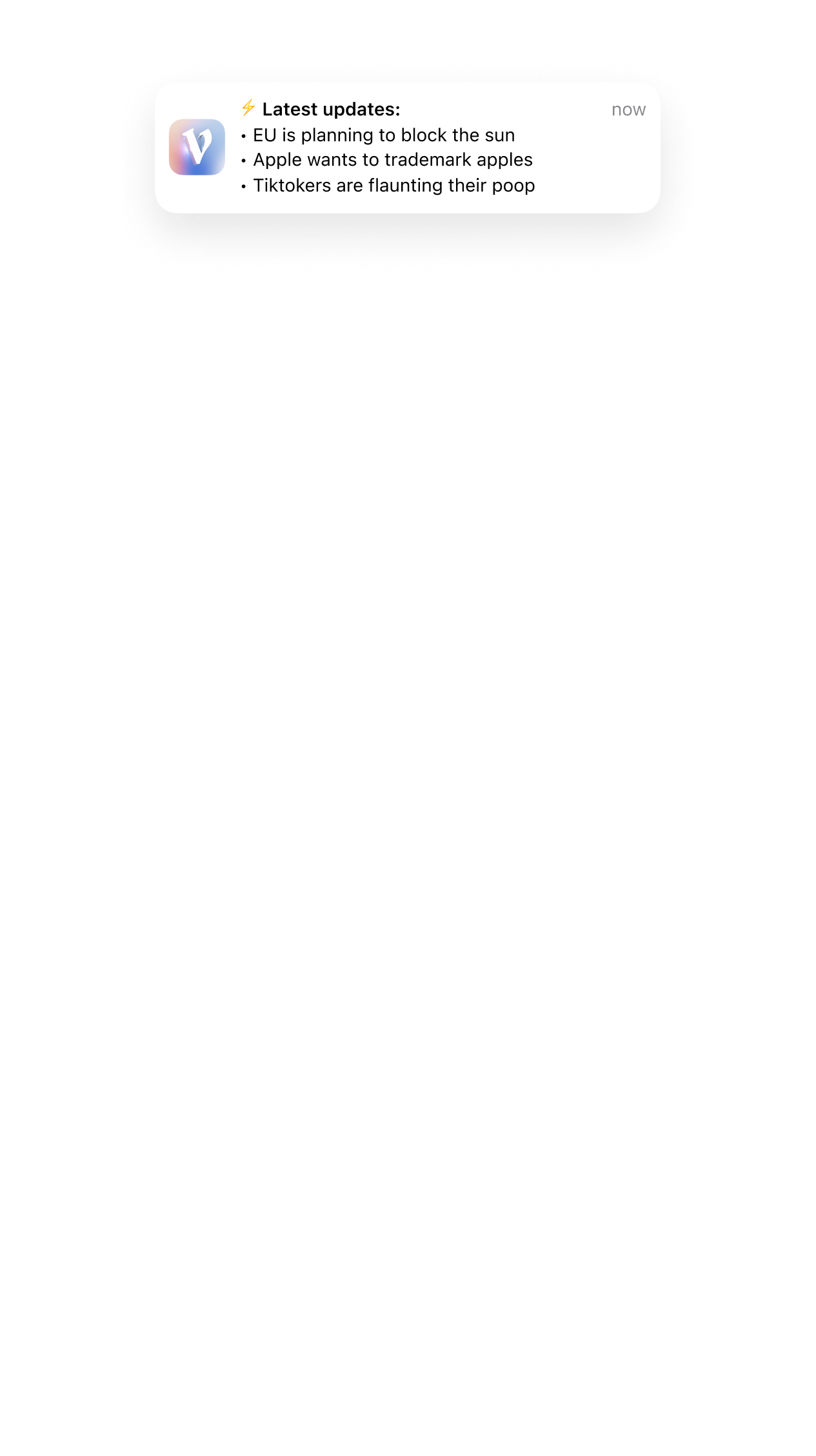Here is a cleaned-up and detailed caption for the image:

"A small cropped screenshot features the section titled 'Latest Updates' in bold black text at the top. To the left of this title, there is a lightning bolt icon, and to the right, the word 'Now' is displayed. Below the title is a bullet point list with three items: 'Planning to block the sun,' 'Apple wants to trademark apples,' and 'TikTokers are flaunting their poop.' Adjacent to the list, on the left, is a logo consisting of a white letter 'V' with a pink-to-blue gradient square as its background. The overall background of the image is white."